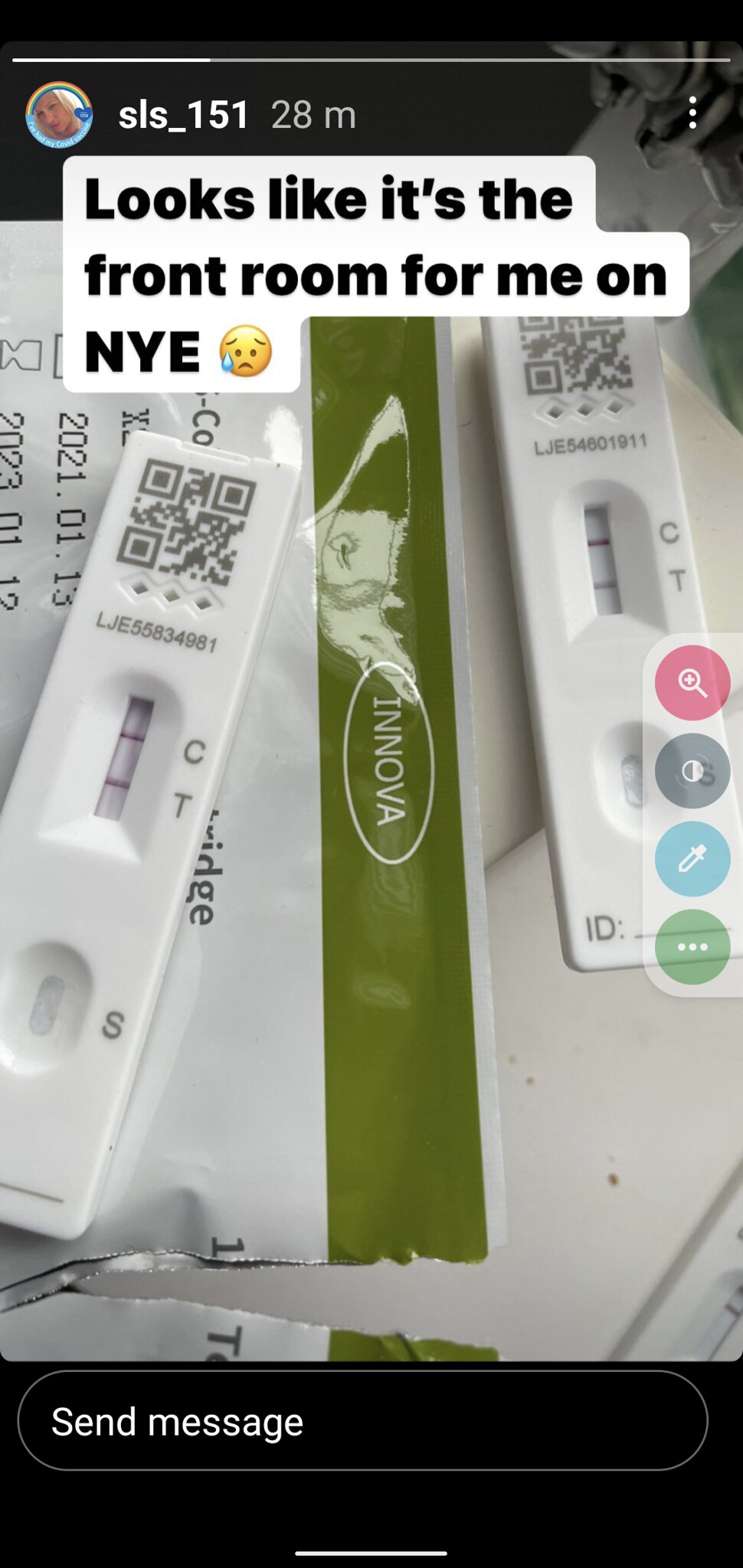This image is a screenshot from a social media reel or story, formatted in the shape of a phone screen. The focus comprises both text and visual elements. At the top, within a white speech bubble with black text, it reads: "Looks like it’s the front room for me on NYE," followed by a sad face emoji with a tear. 

In the main section of the image, there is a receipt at the bottom, dated "2021.01.03." Above the receipt, two used pregnancy tests are displayed side by side, along with their torn packaging. The packaging is green, featuring a circle with the word "Innova" on it. Each white pregnancy test prominently shows two parallel lines, signaling positive results, alongside QR codes at the top. The indicators "C" and "T" are also visible next to the lines on the tests.

At the very top of the screenshot, part of the social media platform's interface is visible. It displays a profile icon of a blonde girl, the username "SLS_151," the timestamp "20 minutes ago," and three dots on the right-hand side indicating additional options. At the bottom of the screen, there is a black box with the option to "send message."